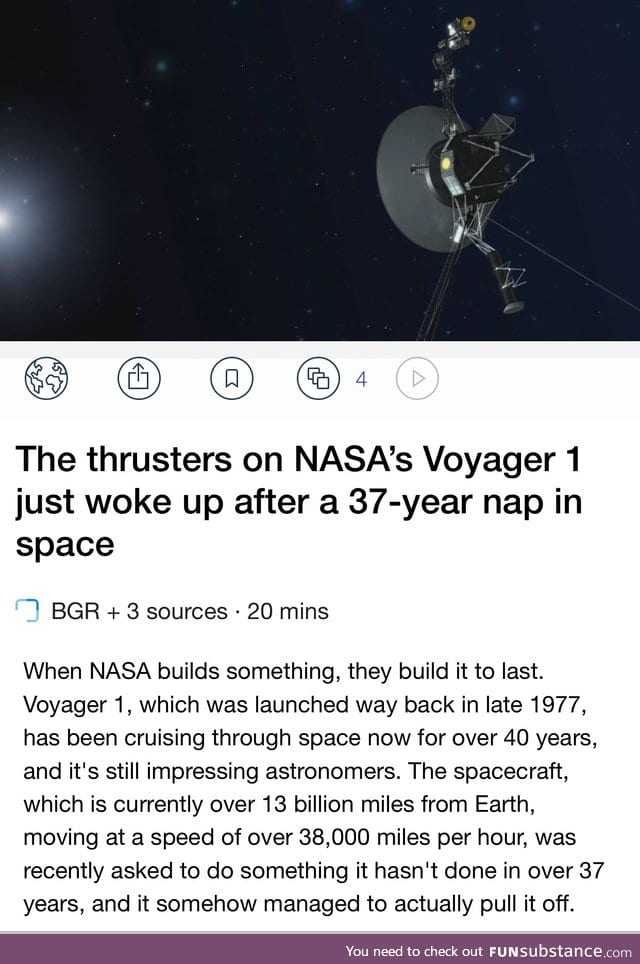The image showcases a screenshot of an article from an online news website, likely a journalistic source. The upper portion of the article features a striking image of a satellite gliding against the vast backdrop of space, with a faint, distant star shimmering on the left side of the frame.

Beneath the image, a series of symbols are arranged horizontally: an Earth symbol, a share/upload icon depicted as a square with an upward-pointing arrow, a bookmark symbol, a copy symbol represented by three stacked squares, the number four, and a play button.

The headline of the article, positioned below the symbols, reads: "The Thrusters on NASA's Voyager 1 Just Woke Up from a 37-Year Nap in Space." Following the headline, the article credits BGR and three additional sources, and indicates an estimated reading time of 20 minutes.

The body text begins as follows: "When NASA builds something, they build it to last. Voyager 1, which was launched way back in late 1977, has been cruising through space now for over 40 years, and it's still impressing astronomers. The spacecraft, which is currently over 13 billion miles from Earth, moving at a speed of over 38,000 miles per hour, was recently asked to do something it hasn't done in over 37 years, and it somehow managed to actually pull it off."

At the bottom of the screenshot, there's a purple footer bar featuring the text "you need to check out funsubstance.com," aligned to the right in white font.